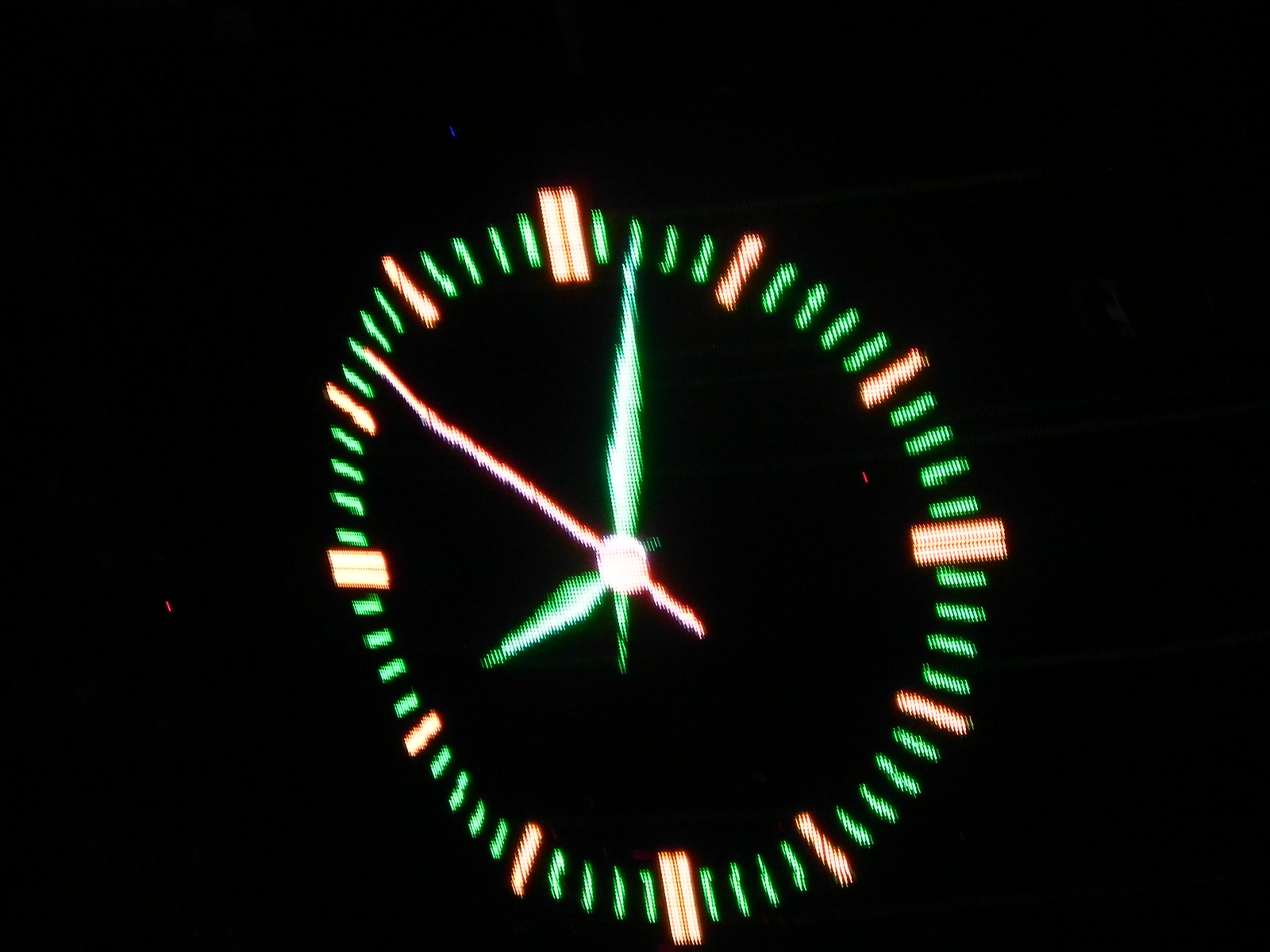This close-up photograph captures a slightly warped analog clock displayed on a digital screen, set against a black background that emphasizes the pixelation. Central to the image is a circular clock face devoid of any numbers or labels, comprised entirely of hash marks in varying colors. The larger hash marks, indicating the quarters (12, 3, 6, and 9), are orange, and they alternate with sets of smaller green hash marks. The pattern around the clock includes sequences with two orange marks close together, followed by four green marks, then a singular orange mark, and repeating. At the heart of this clock face are three hands: two green hands showing the hour and minute, pointing left and right respectively, and a longer red hand for the seconds. A small red dot is visible near the bottom-left corner. The time displayed on the clock reads approximately 8:02. The detail of these features, along with the digital nature of the display, creates an intricate and visually engaging image reminiscent of both a speedometer and a traditional clock.